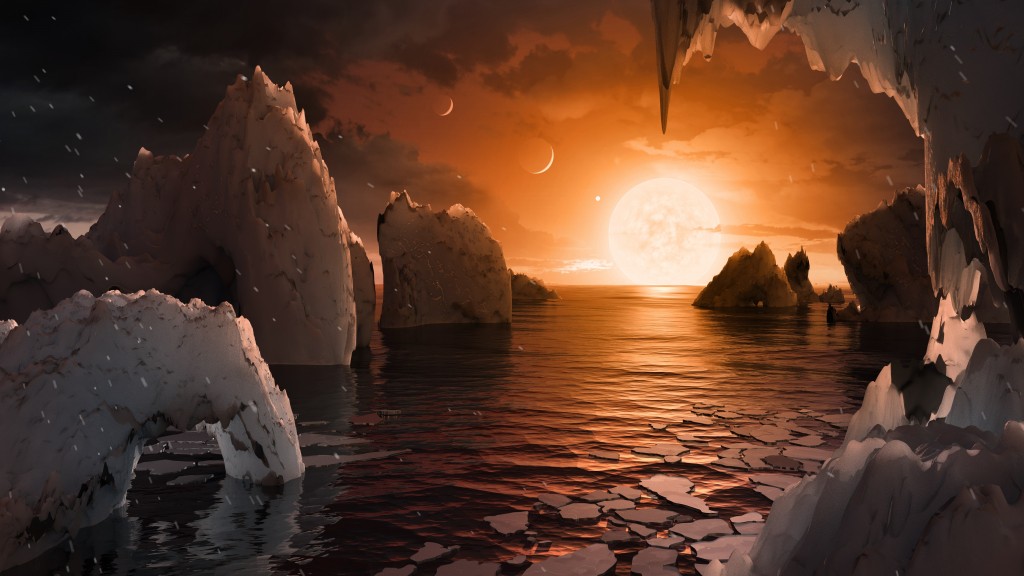This digital artwork portrays a dramatic, fantasy-style seascape on what appears to be an alternative planet. The scene is dominated by a dark, apocalyptic atmosphere, characterized by a color palette of black, gray, and orange. The expansive ocean is dotted with jagged rock formations and iceberg-like structures, giving an impression of an arctic landscape. Sheets of ice float on the water's surface, contributing to the film noir, moody aesthetic of the piece. 

Looking towards the horizon, a large, brightly lit white planet, reminiscent of the Sun, hangs low, suggesting either sunrise or sunset. Flanking this main celestial body are two smaller planets or moons, adding to the otherworldly feel. The overcast sky is thick with dark and cloudy formations, enhancing the scene's enigmatic mood. On the right side of the image, a pronounced jagged rock overhangs, creating a cave-like structure. The distant galaxy of stars completes the ethereal and haunting atmosphere of this intricately detailed piece.